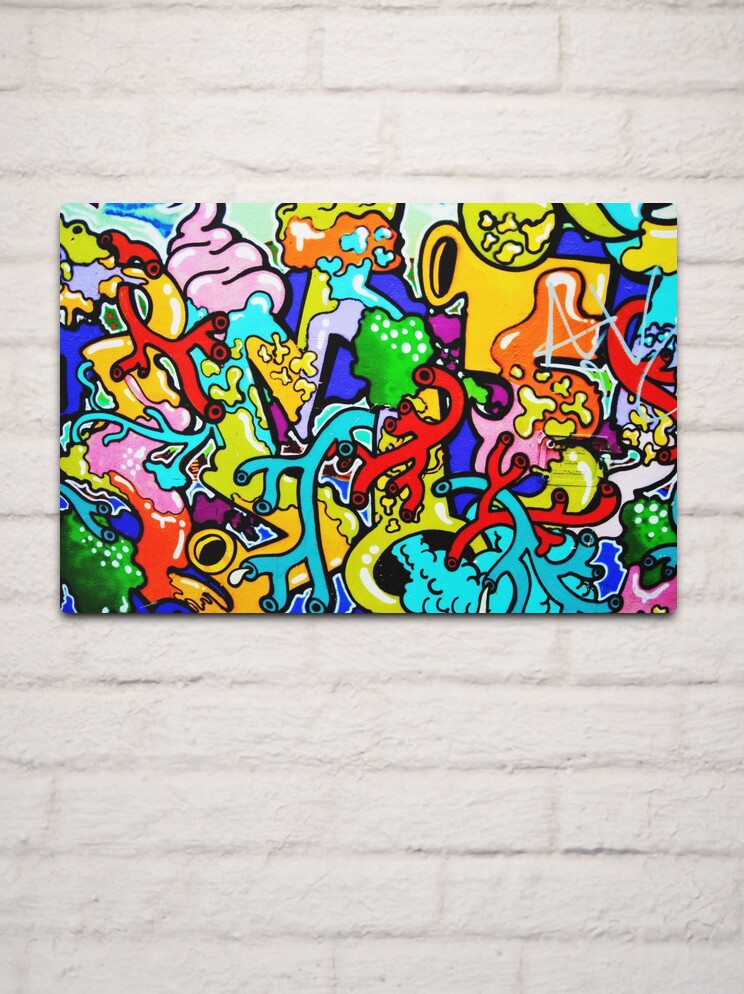This photograph captures a vivid, abstract painting hanging on a white-painted brick wall. The rectangular canvas, unframed, is a modern art piece likely executed with acrylics. The artwork is a bold, vibrant collection of colors and shapes, predominantly featuring bright, poppy hues such as green, red, orange, pink, purple, blue, and gold, all richly pigmented and highlighted with specks of white. The composition suggests an underwater theme with elements resembling coral reefs and sea cucumbers, but also alludes to internal body structures like veins, capillaries, and heart valves. The abstract forms include branching tubular structures in red and blue, thicker gold-colored pipes, and liquid-like blue areas. The painting’s exaggerated, cartoony style with intricate black line art creates a visually striking and non-realistic assemblage, making it an engaging piece of modern art. Notably, there is no visible text or signature on the artwork.